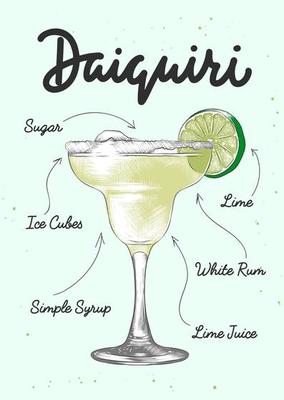The image is a detailed, hand-drawn sketch of a daiquiri recipe, set against a pale mint green background. At the top, in bold black cursive, the word "daiquiri" is prominently displayed. The sketch features a classic margarita glass filled with a green daiquiri, complete with a slice of lime on the rim. Various ingredients are labeled with arrows pointing to their respective parts of the drink, including sugar on the rim, ice cubes at the top, simple syrup, lime juice, and white rum. The drawing, designed to resemble a colored pencil sketch, appears digitally created with a script-like font for the labels. This image serves as a quick and easy-to-follow reference guide for making a daiquiri, perfect for platforms like Pinterest.